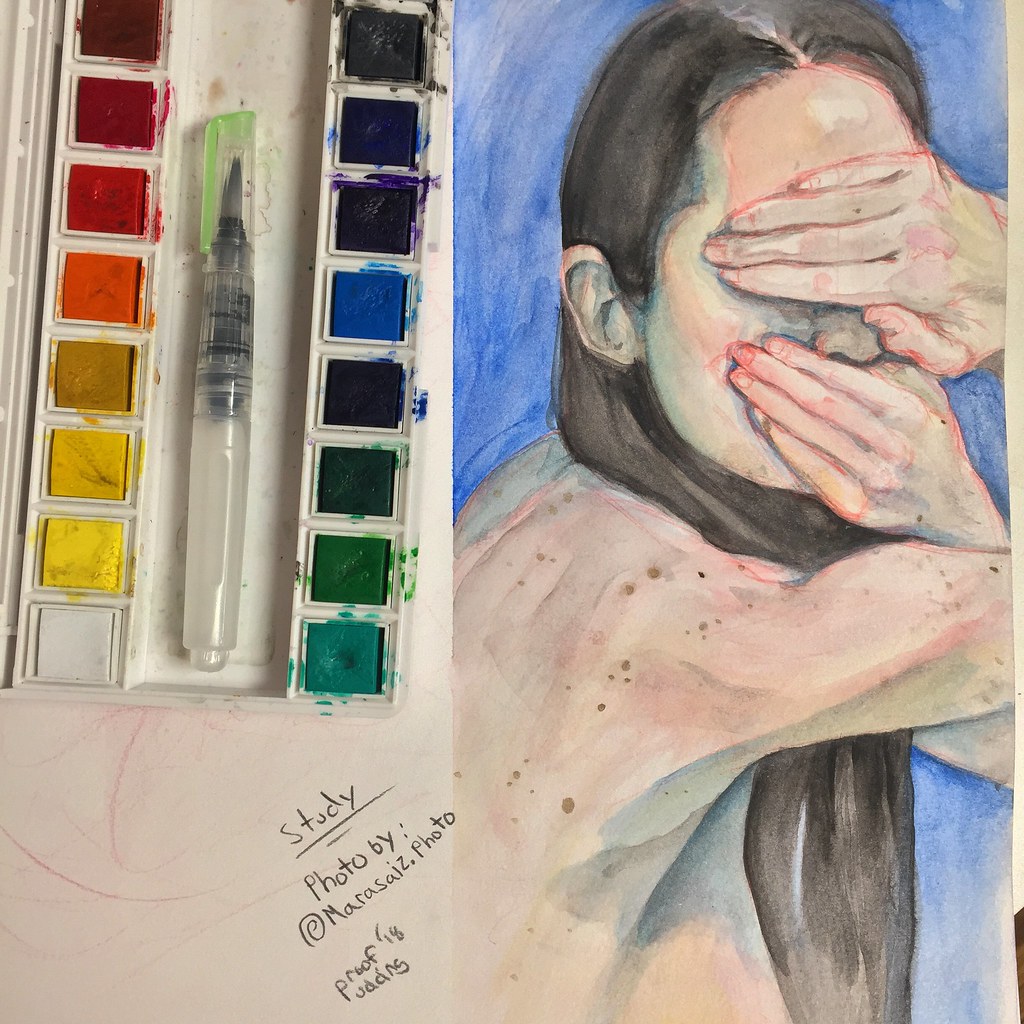This detailed watercolor illustration presents a haunting image of a young woman with long, dark black hair, and light, freckled skin, appearing emaciated and showing a frail back. Her hands are raised, covering her eyes and mouth, suggesting a sense of concealment or distress. The background is painted in a wash of blue, contrasting with her pale skin and dark hair. The painting is accompanied by a white container of watercolor paints situated to the left, featuring an assortment of smeared colors: reds, oranges, yellows on one side, and blues, greens on the other, showing signs of recent use. A small watercolor brush with a white plastic handle and a green cap lies amidst the paints. At the bottom of the image, partially obscured text reads "study photo by @MaraSize.photo", dated approximately 2018. The combination of the watercolor detailing, the emotional subject matter, and the scattered painting tools evokes a poignant, artistic narrative.